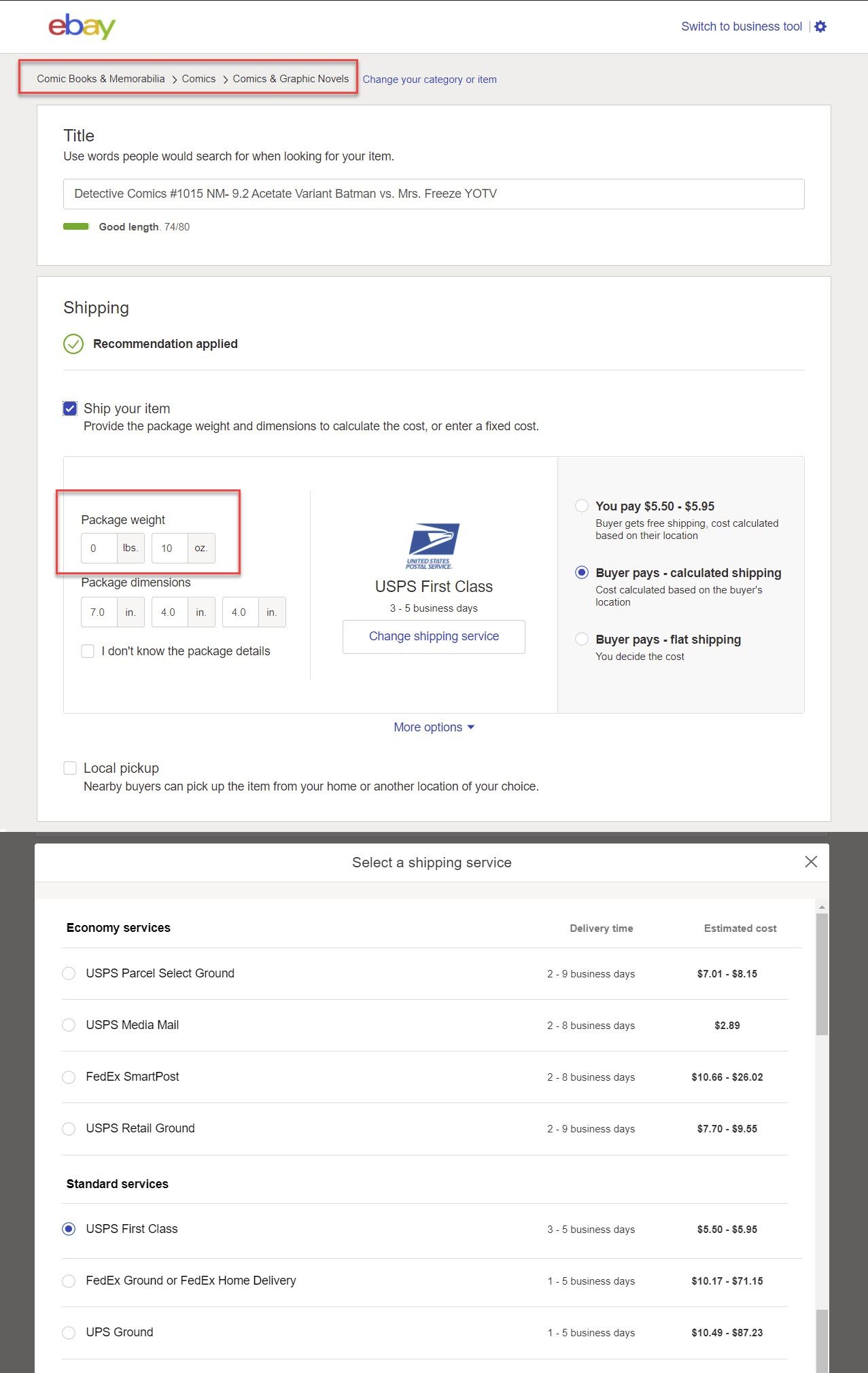This screenshot from the eBay website captures a listing creation page with a focus on comic books and memorabilia, specifically an Aero comics category. At the top left, the iconic eBay logo is prominently displayed, with each letter in a different color: red 'e', blue 'B', yellow 'a', and green 'y'. To the top right, there's an option to switch to the business tool.

Outlined in a red rectangle is the section for selecting categories, specifically, "Comic Books and Memorabilia > Aero Comics > Aero Comics & Graphic Novels," with an option to change the category or item.

The listing title reads: "Detective Comics #1015 NM-9.2, Ace Tate Variant Batman vs. Mrs. Freeze, YOTV." This descriptive title adheres to eBay’s recommendation to use searchable keywords. 

The shipping section is detailed and comprehensive. The recommended shipping parameters are highlighted, with a package weight of 0 pounds and 10 ounces, enclosed in a red rectangle. The package dimensions are specified as 7.0 inches in length, 4.0 inches in width, and 4.0 inches in height. An unchecked box below notes an option for users who are unsure of the package details.

USPS First Class shipping, which takes 3-5 business days, is selected. Above this option, the USPS logo, featuring an eagle in white against a blue background, is visible. Three radio buttons provide different shipping cost options:
1. Seller pays ($5.50-$5.95) with free shipping for the buyer.
2. Buyer pays calculated shipping based on their location (selected).
3. Buyer pays flat shipping rate set by the seller.

Additional shipping options include:
- Local pickup for nearby buyers.
- Economy Services: 
  - USPS Parcel Select Ground (2-9 business days) at $7.01-$8.15
  - USPS Media Mail (2-8 business days) at $2.89
  - FedEx SmartPost (2-8 business days) at $10.66-$26.02
  - USPS Retail Ground (2-9 business days) at $7.70-$9.55
- Standard Services:
  - USPS First Class (3-5 business days) at $5.50-$5.95 (selected)
  - FedEx Ground or Home Delivery (1-5 business days) at $10.17-$71.15
  - UPS Ground (1-5 business days) at $10.49-$87.23

This detailed breakdown ensures clarity in listing and shipping options for potential buyers.